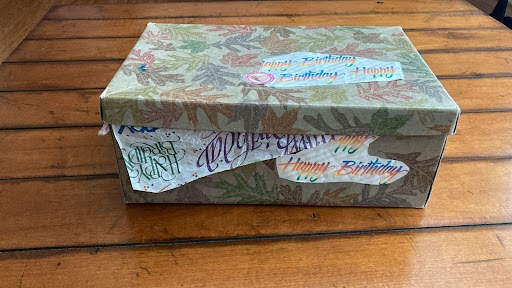The image depicts a small gift box, resembling the shape of a standard shoebox, resting on a wooden table with a lighter brown color and occasional dark brown streaks. The box is covered in decorative paper featuring an array of colored leaves in shades of blue, orange, yellow, and green, presenting a fall-like theme. Adorning the box are multiple "Happy Birthday" messages: a blue sticker with rainbow writing on the top right, another sticker on the side, and crepe paper with the same message partially hanging out from the edge. The overall presentation of the box appears simple and homemade, suggesting it is a thoughtfully yet modestly crafted birthday gift.